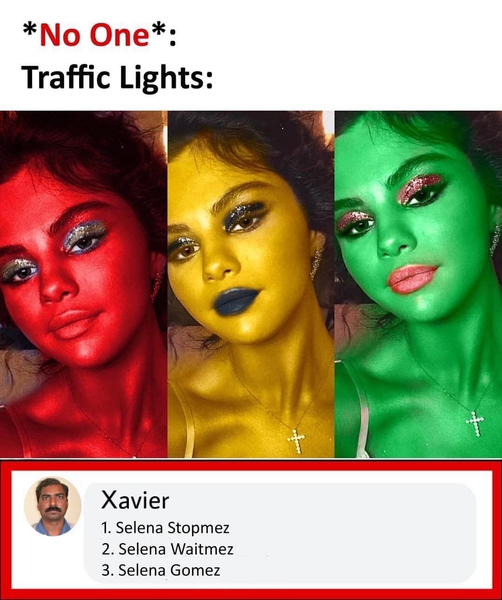This image appears to be a social media post designed for humor, featuring a witty play on traffic lights and the celebrity Selena Gomez. At the top of the image, in red text with asterisks on either side, the phrase "No one" is written, followed by the words "traffic lights" in black text. Directly beneath this are three identical images of Selena Gomez, each altered in color to resemble a traffic light: red, yellow, and green. Her skin is tinted to match the respective colors, emphasizing the theme.

Each of these images of Selena Gomez, which are equal in size and aligned side-by-side, associates her with the corresponding traffic signal colors. Further, beneath these images, there is additional text and the image of a man, presumably named Javier, who is identified by a headshot featuring a Mediterranean appearance, short hair, thick eyebrows, and a bushy mustache, while dressed in a blue shirt.

The text at the bottom humorously labels the traffic-light-themed images of Selena Gomez in alignment with their colors: "1. Selena Stopmez" for the red-tinted image, "2. Selena Waitmez" for the yellow-tinted image, and "3. Selena Gomez" for the green-tinted image. Each label cleverly correlates with the conventional traffic light signals - Stop, Wait, and Go. The entire setup, from text to images and their playful descriptions, suggests the post is crafted for social media engagement, drawing on visual humor and wordplay.